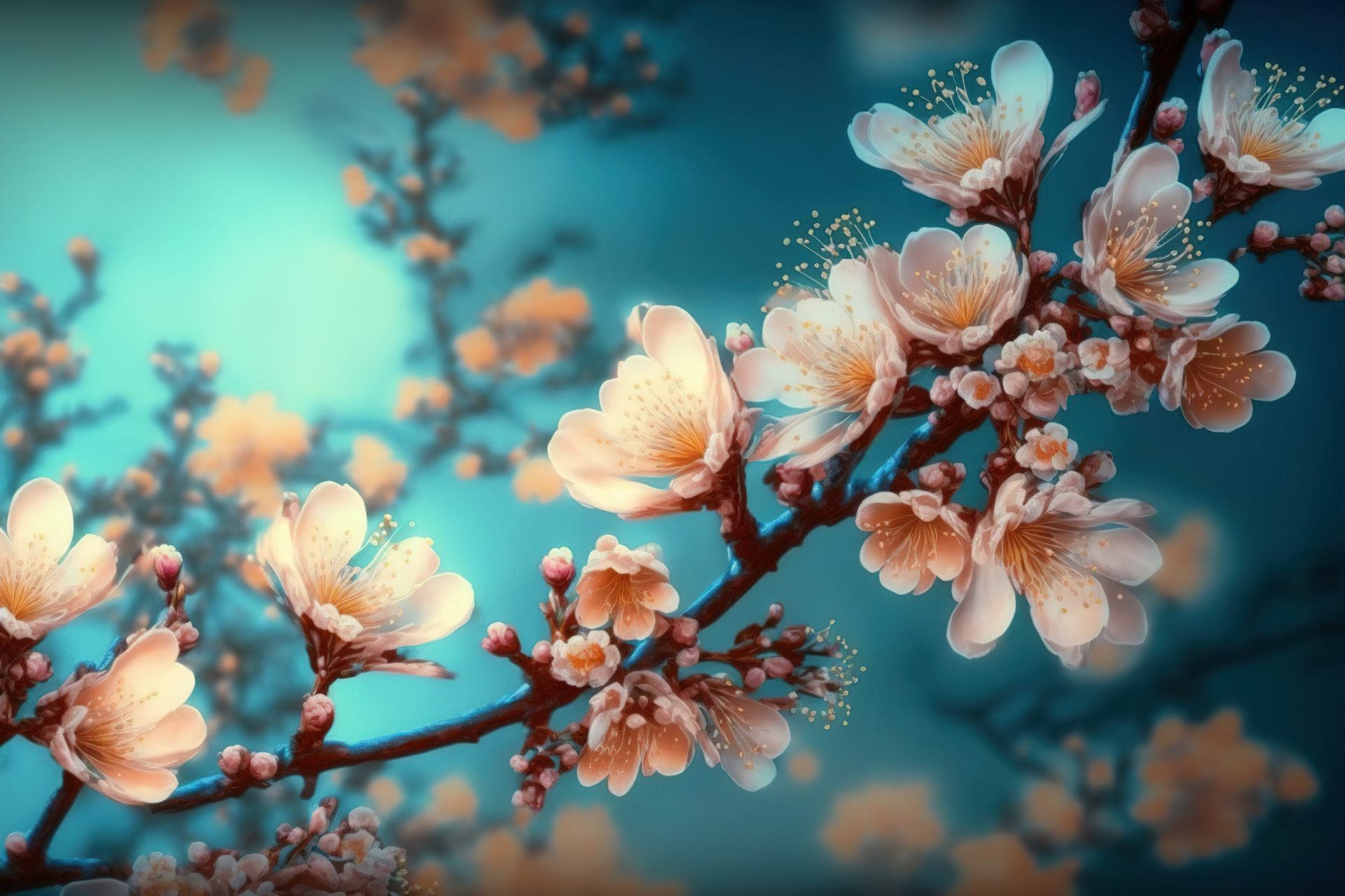This artwork, likely either a painting or a computer illustration, captures the intricate beauty of a tree branch adorned with flowers. The main branch, colored a rich brown, emerges from the lower left corner of the image and ascends gracefully to the upper right. It is heavily dotted with delicate flowers, predominantly in shades of light pink and white. These blooms are a mix of fully open flowers and smaller buds, with thin filaments and white stamen prominently visible, hinting at their readiness to pollinate. The flowers boast centers in shades of orange and yellow. A blue backdrop, reminiscent of a sky or possibly an underwater scene due to its aqua hue, enhances the visual appeal. The background features blurred outlines of additional limbs and an indistinct mix of colors, with notable blue and orange blurs in the lower right corner. The intersection of detailed foreground and abstract background elements creates a compelling visual narrative, making the viewer ponder the true setting of this floral display.